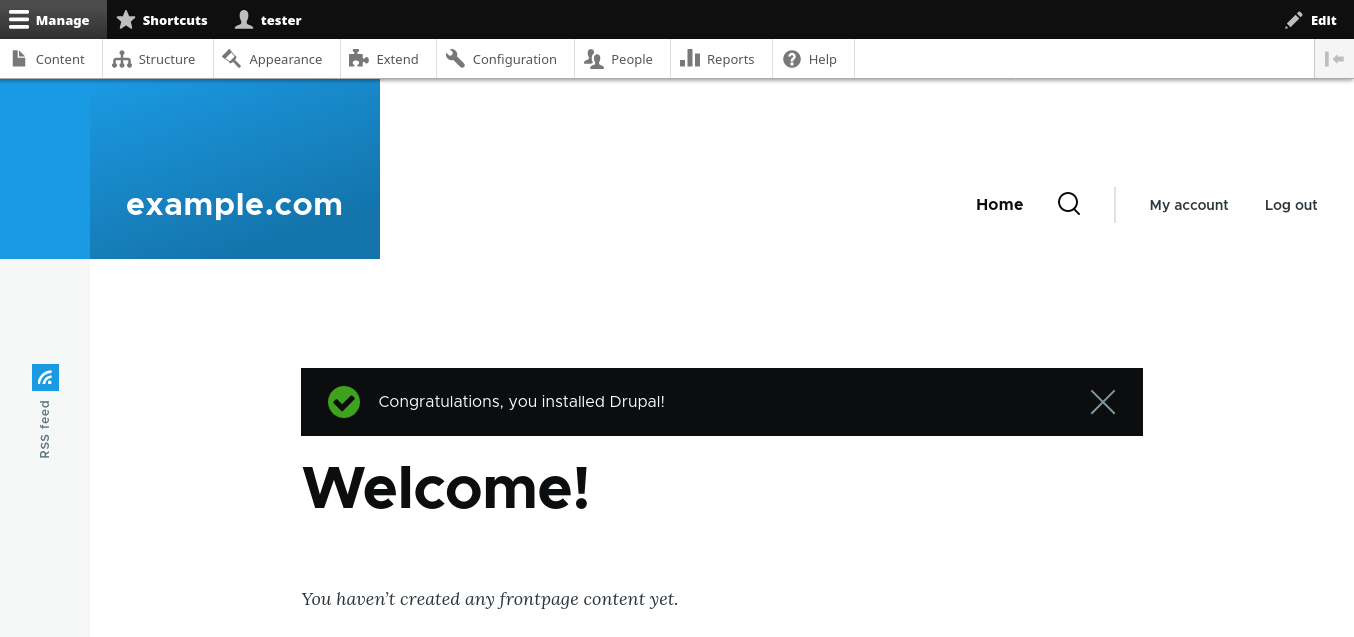The image is a horizontally rectangular screenshot of a website interface showing the successful installation of Drupal at example.com. The top section features a black horizontal banner with "Manage Shortcuts" and "Tester" buttons on the left, and an "Edit" button on the right. Underneath, there is a narrow white horizontal banner with additional options listed from left to right: "Content," "Structure," "Appearance," "Extend," "Configuration," "People," "Reports," and "Help."

On the left side beneath this second banner is a small blue horizontal rectangle that contains the text "example.com" in white. Opposite this blue box, on the right side, are options for "Home," "Search," "My Account," and "Log Out." Dominating the center of the frame is a black horizontal rectangle featuring a green circle with a black check mark inside it. To the right of the green circle, white text reads, "Congratulations, you installed Drupal."

Below this congratulatory message on a white background, the word "Welcome!" is displayed prominently, followed by a smaller message indicating, "You haven't created any front page content yet."